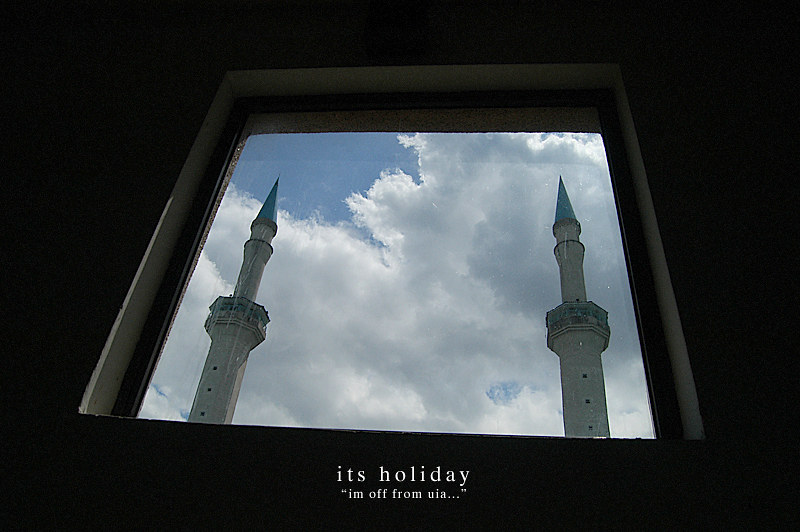The photograph captures a scene from inside a room, looking out through a window with a white windowsill and a black frame. Below the window, in white letters, is the caption "It's holiday." Beneath that, in smaller white text enclosed in quotations, it says, "I'm off from UIA...". The exterior view showcases a blue sky with white clouds and two tall towers, each topped with a pointed, cone-shaped blue spire. The towers have a white base and appear to feature three vertically aligned windows or elements resembling a balcony, detailed in blue and white. There are no people in the image, and the photograph is unsigned.